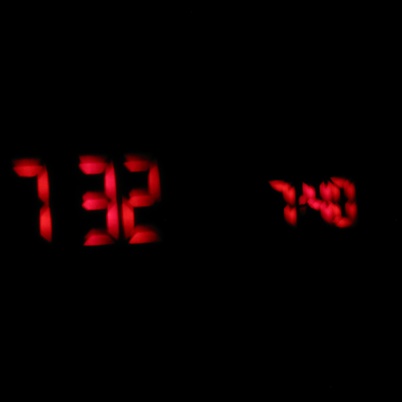This photograph features a pair of vivid neon red digital numbers on a predominately black background, reminiscent of old-style LED displays found on alarm clocks from the 80s or 90s. Spanning horizontally across the center of the image from left to right, the numbers "732" appear prominently on the left and "740" on the right. Despite the slight blurriness and out-of-focus edges, the numbers remain clearly legible. There is no colon between the digits to indicate time, enhancing the ambiguity of what these numbers represent. The equal distribution of black space above and below the numbers adds to the symmetrical composition of the photo.